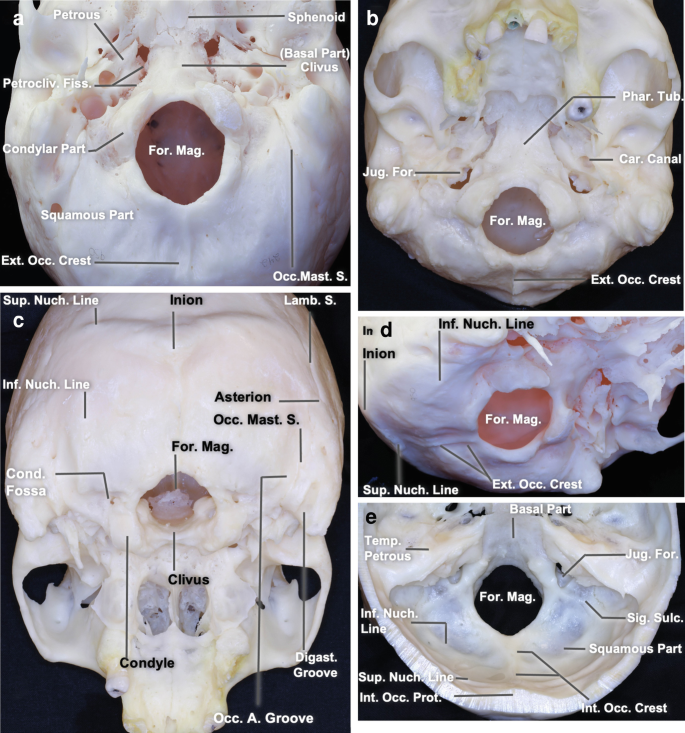The image is a detailed collage of five annotated photographs of skull components arranged in a rectangular shape, roughly five inches high and four to five inches wide. Each photograph, taken against a black background, is labeled with letters A through E. In the top-left corner (A), the skull displays labels such as "Petros," "Squamous Part," "Sphenoid," among others, with lines pointing to the corresponding anatomical areas. Below it, in the lower-left corner (B), another image labeled "ext. oc. crest," depicts detailed parts like the "Sphenoid" and "Basal part clevis." 

On the right side, the central photograph (C) features the skull's base, with annotations such as "Jug4," "Formag," "Car. Canal," and "Condyle." The lower right image (D) is marked with "Cond. Fossa," "Sup. Nuc. Line," and "Inferior Nuclear Line," among others, giving a comprehensive view of the detailed labeling. Lastly, in the upper right-hand corner (E), the skull showcases labels like "Temporus Petreus" and "Squamous Part," with intricate annotations pointing to each specified area. This meticulously labeled collage collectively provides an in-depth anatomical reference of various skull features from different perspectives.